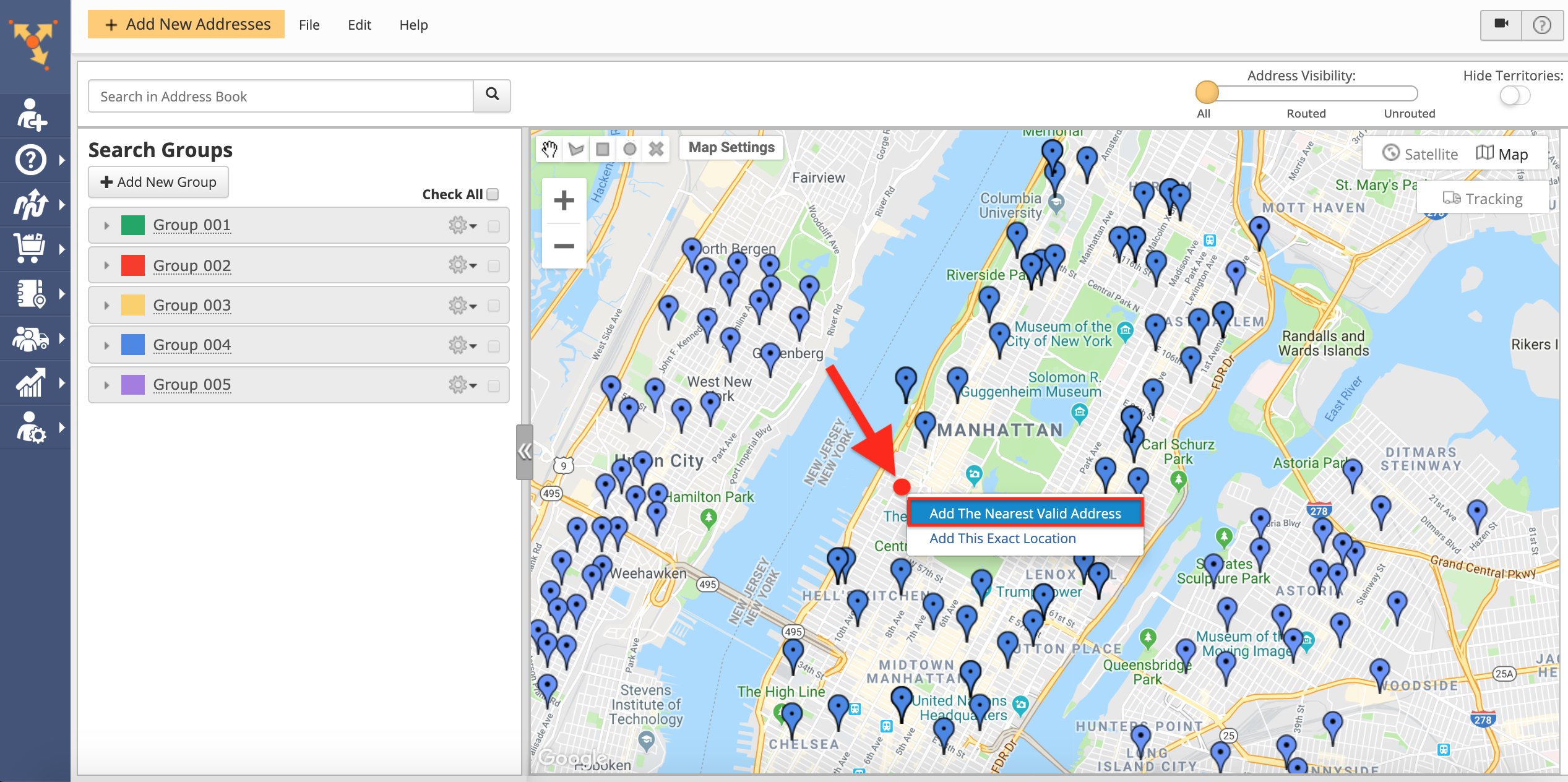This image is a screenshot of a web page displayed in landscape mode, primarily featuring a map centered on Manhattan with surrounding areas also visible. The map, which occupies about two-thirds of the image starting from the right, showcases several tagged locations. These tags are marked by blue circles with a central dot and an arrow pointing downwards. 

Prominently in the center of the map, where Manhattan is located, there's a blue text box containing the instruction: "Add the nearest valid address." This text box is highlighted with a red border. Above it, in the top left corner, there's a small red circle which is pointed out by a red arrow originating from the adjacent landmass next to Manhattan.

On the far left side of the screenshot, there's a vertical column with a blue background displaying various icons and arrows in white. Adjacent to this column are the words "Search groups," followed by a clickable tab labeled "+ Add new group." Below this, there's a list of groups, each prefixed by "Group" and a numeric identifier. Group 001, highlighted with a green box to its left, is at the top of this list. Subsequent groups are color-coded and listed in order: Group 002 in red, Group 003 in yellow, Group 004 in blue, and Group 005 in lilac.